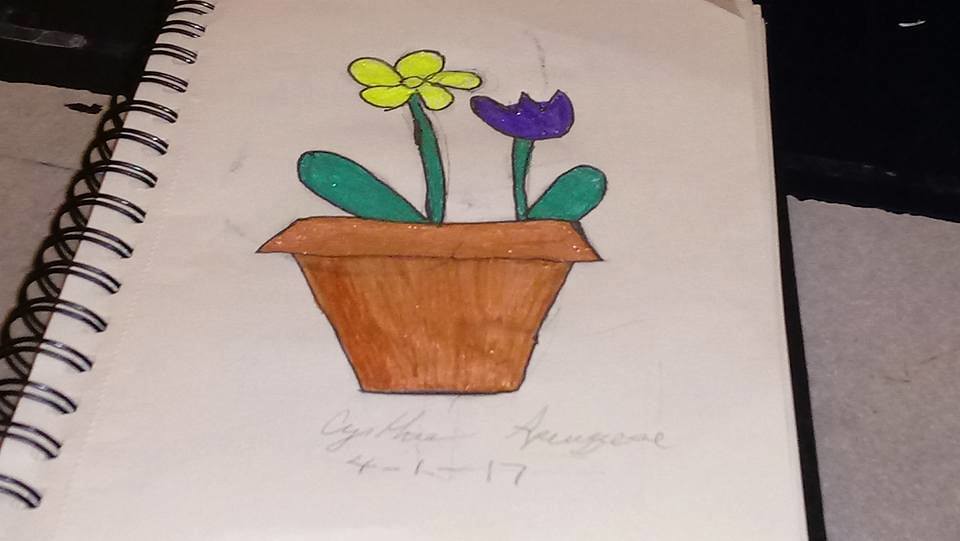In the image, there is a hand-drawn illustration of a flowering plant captured on white paper within a black ringed notebook. The plant is depicted in brown, having two distinct flowers. The first flower on the left side features five petals and is associated with a green leaf, while the second flower on the right side resembles a purple lily, also accompanied by a green leaf. The drawing is simplistic yet charming, with minimal detailing, capturing the essence of the plant. At the bottom of the illustration, there is a cursive signature that appears to start with a "C" and possibly reads "Cynthia," with a last name beginning with "A" and ending in "E." The drawing is dated 4-1-17, indicating it was created on April 1st, 2017.